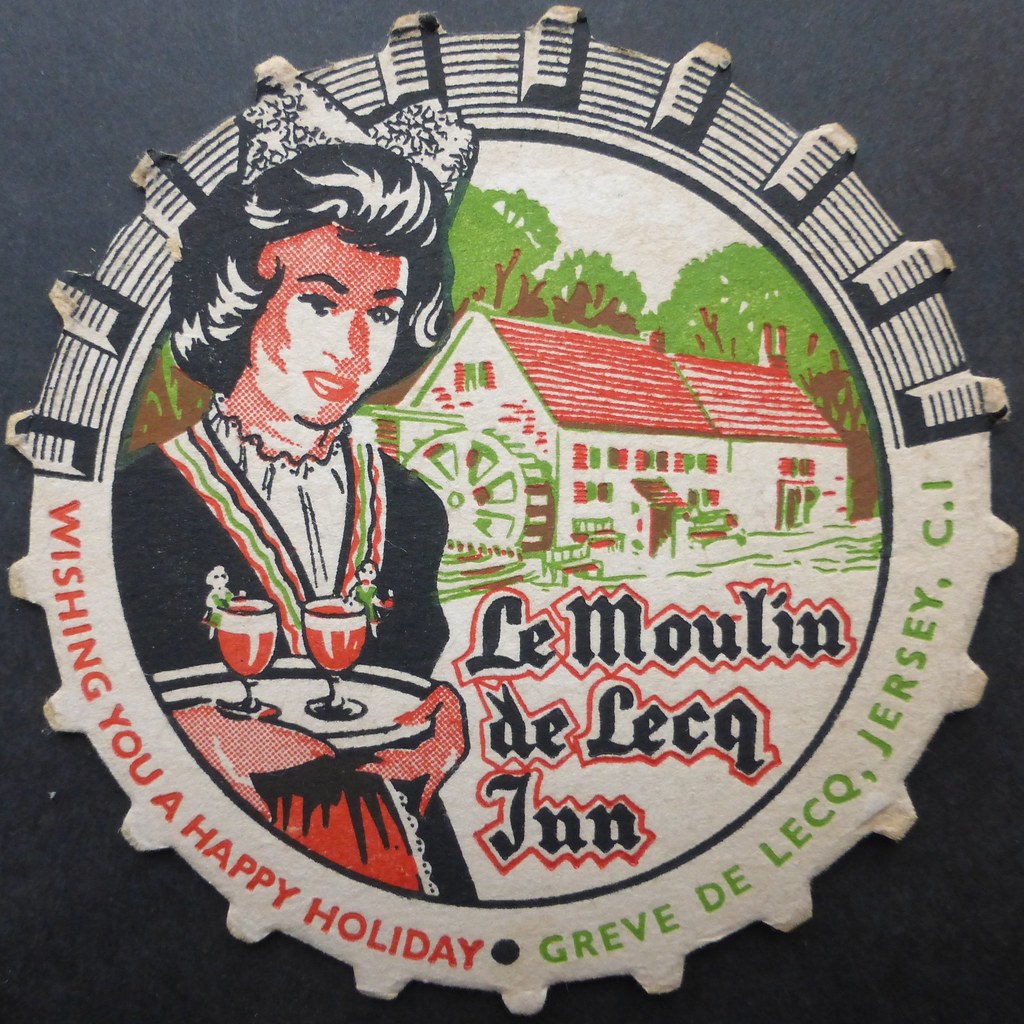The image depicts a holiday greeting from Le Moline de L'Eca Inn in Greve de Lec, Jersey CI. It is set against a black background and primarily features a circular design with spiked edges, resembling a wheel, nearly touching the edges of the photograph. Within the circle, an old-fashioned-looking woman positioned to the left is wearing a dark blouse, a dress, and a red apron with a bow in her hair. She is holding a tray with two cocktails in front of her. To her right, there is a depiction of a house with a wheel beside it and some trees above it. The top half of the circular design includes several stripes, while the bottom half features text in red and green fonts. In red lettering along the edge of the circle, it says, "Wishing you a happy holiday," and in green, it reads "Greve de Lec, Jersey CI." The overall theme and style of the image suggest a joyful holiday message from a restaurant or bar.